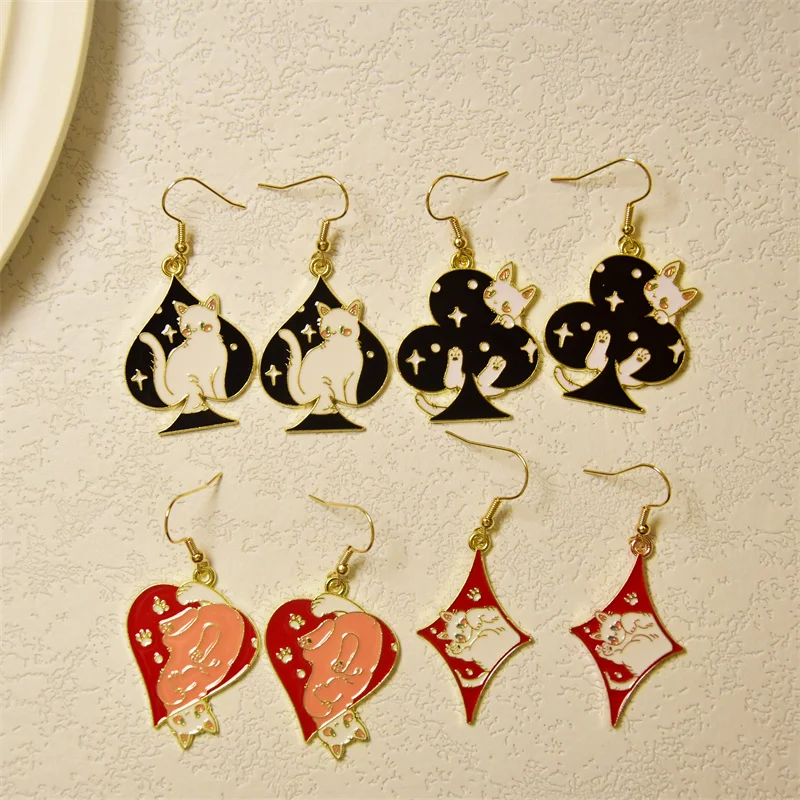This compelling photograph depicts a thoughtful layout of four distinct sets of earrings presented against a white textured background. Each set embodies a unique interpretation of card suits with an accompanying whimsical cat motif, suggesting a harmonious theme likely created by a single artist. In the top row, the left pair showcases black spades with an endearing white cat sitting prominently in the middle, overlapping the edges to infuse a sense of playfulness. Next to it, the black clubs feature a cat curiously peering out, only visible by its head and feet, adding a touch of mystery and charm. The bottom row transitions to vibrant red hues; the left pair illustrates red and pink hearts with an upside-down cat clinging tenaciously to the shape, and the pair on the right displays a red diamond, within which a white cat is gracefully curled. Each earring set is meticulously crafted with golden hooks, underscoring both elegance and attention to detail. This cohesive collection beautifully merges themes of card suits and endearing feline antics, captivating viewers with its artistic and playful essence.